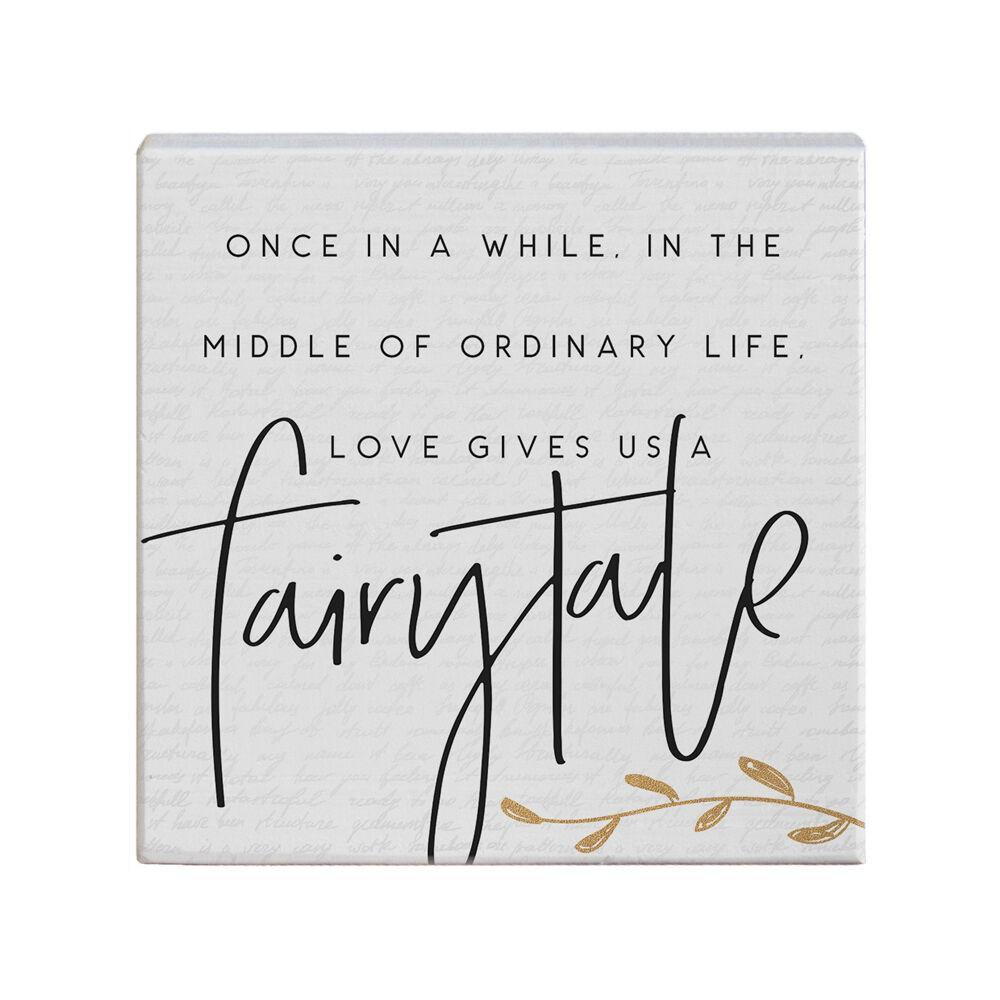The image depicts a perfectly square, thin white box set against an equally white background, making it appear as if it's floating. Measuring roughly four inches per side, the box features centered black text in all capital letters spread over three lines: "ONCE IN A WHILE IN THE," "MIDDLE OF AN ORDINARY LIFE," and "LOVE GIVES US A." Following this, in a large, stylized cursive font occupying almost half the box, is the word "fairytale," written in lowercase. To the bottom right of "fairytale," there's a subtle golden-brown vine with leaves extending from the center toward the right edge of the box. Additionally, the white background behind the box has faint, barely readable silver cursive text, giving a textured impression upon closer inspection. The overall impression is that of a delicately designed gift, possibly containing an unknown surprise, encapsulating the notion that "once in a while in the middle of ordinary life, love gives us a fairytale."